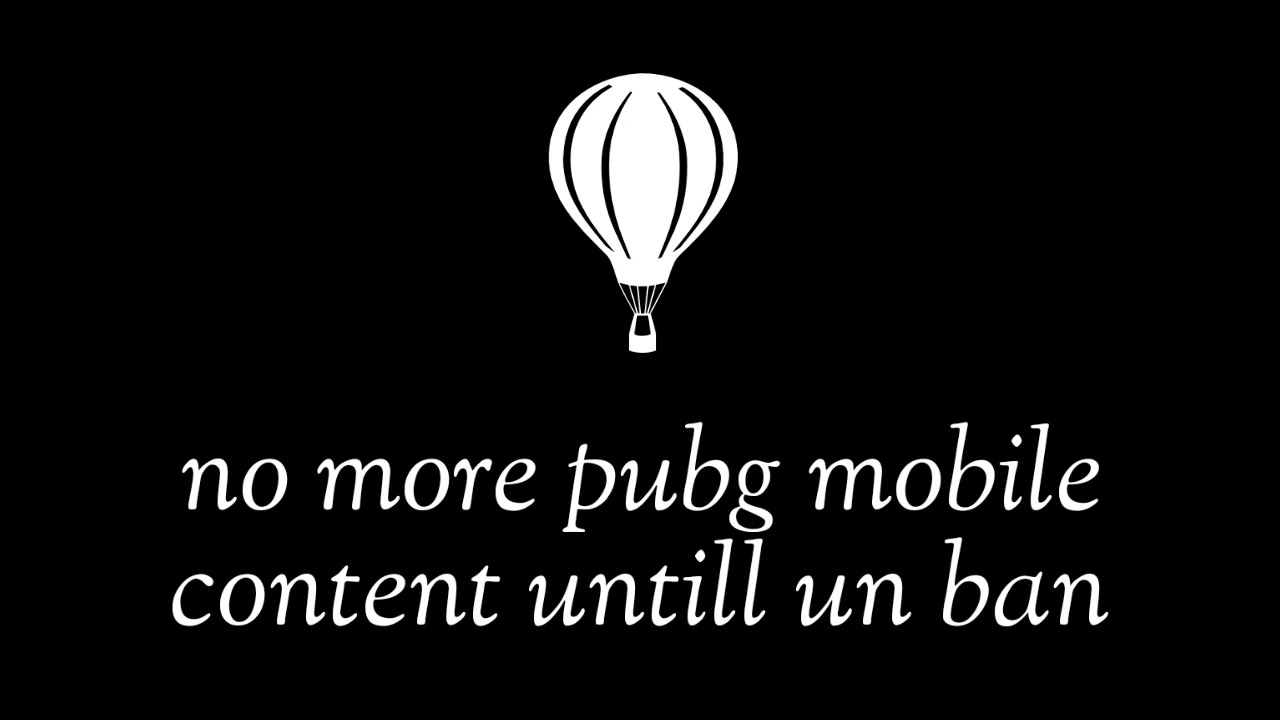The image portrays a clear statement against a flat, purely black background. Dominating the upper center is a detailed white emblem of a hot air balloon with a hanging basket, devoid of occupants. Rendered in white cursive text on the bottom half are two lines expressing a sentiment of protest: the first line reads "no more P-U-B-G mobile," and the second line, slightly larger and featuring a typographical error in lowercase letters, states "content until unban," with 'until' misspelled as "untill" and 'unban' written as "U-N ban." The combined imagery and text suggest a social media or community protest likely initiated by a video game player, streamer, or professional gamer, highlighting their intention to cease producing PUBG Mobile content until their ban is lifted. The prominent hot air balloon image adds an emblematic touch to this protest statement.